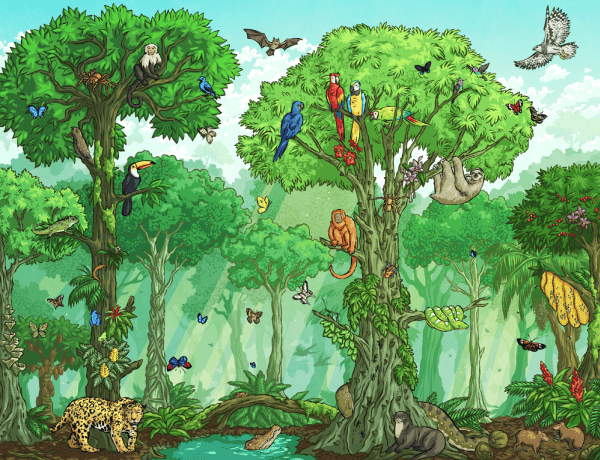In this vividly detailed illustration of a jungle scene, we observe a lush, verdant forest teeming with life. Dominating the landscape are several tall trees with strong trunks, adorned with green leaves and ensnaring vines, their canopies forming a dense cover. Among these trees, a wide variety of wildlife is depicted in their natural habitat. 

In the forefront, on the bottom left, lies a leopard prowling near the roots, with characteristic yellow fur and black spots. To its right, a small body of water, possibly a pond or stream, breaks the forest floor, its serene surface disturbed by a crocodile or alligator with its head emerging from the water. The visual is enriched with various tropical bushes scattered throughout.

The trees are bustling with activity. Numerous colorful birds, including parrots, toucans, and other vibrant species like blue, red, and rainbow-colored birds, perch on the branches or are mid-flight. A green snake is coiled around a branch, and a sloth hangs leisurely from the treetops. Monkeys, in different shades of brown and black, swing from the vines or perch high in the foliage. We also see butterflies flitting gracefully among the trees, adding to the animated atmosphere.

Up in the sky, birds of prey like a hawk glide effortlessly alongside an incongruous bat, despite the daytime setting. Hidden within this panorama, a blue butterfly, a spider, and even a tarantula add to the jungle's rich biodiversity. The lighting suggests sunlight filtering through, casting a gentle glow on the scene, and adding to the vibrant hues of the foliage and wildlife. Altogether, this cartoon-like drawing beautifully captures the essence and abundant life of a thriving jungle ecosystem.